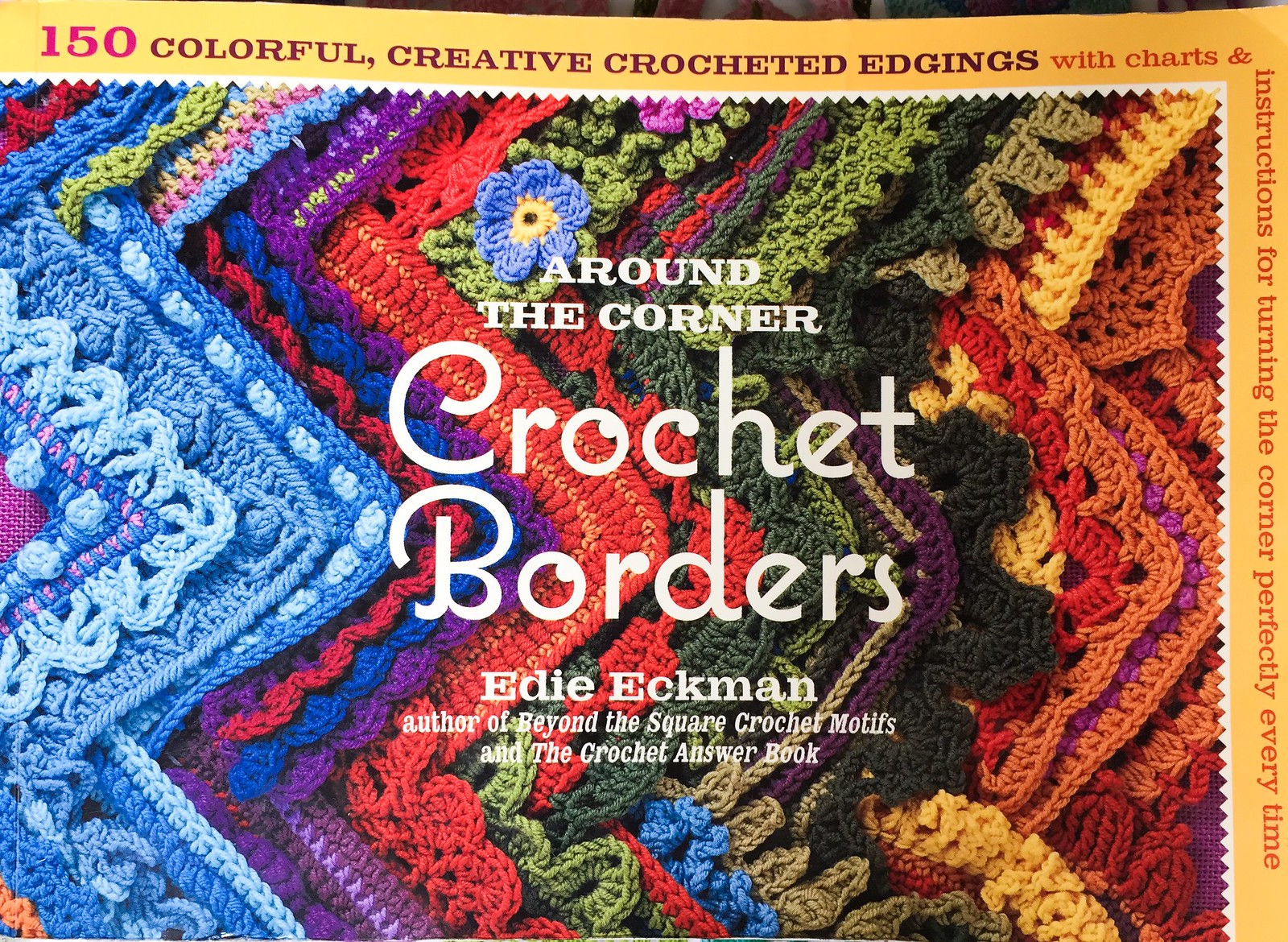The image is a detailed photograph taken from above, showcasing the top half of a crochet magazine cover. Dominating the visual is a bright yellow border that runs along the top and right side, featuring the text: "150 colorful, creative, crocheted edgings with charts and instructions for turning the corner perfectly every time". At the corners, the ampersand is cleverly positioned right at the edge.

The central area showcases a stunning collection of crocheted zigzag designs and various patterns, including vibrant flowers. The palette bursts with numerous shades of blues, reds, purples, oranges, yellows, and greens. These diverse patterns and colors create a rich, textured background.

Overlaid on this colorful tapestry is the prominent title in white text: "Around the Corner, Crochet Borders," followed by the name of the author, Edie Eckman, known for "Beyond the Square, Crochet Motifs" and "The Crochet Answer Book." The layout effectively uses the colorful crochet designs to highlight the instructional and aesthetic appeal of the magazine.